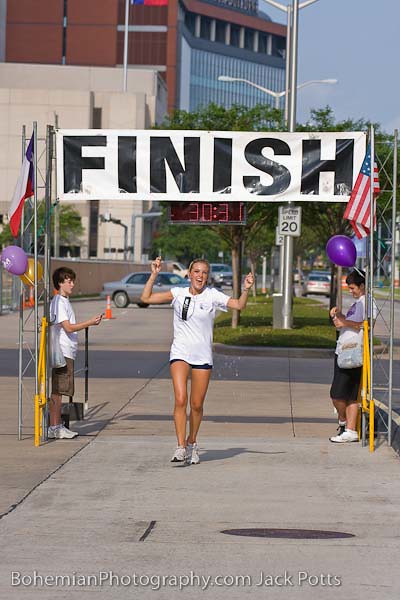In the image, a woman triumphantly crosses the finish line of a race, her arms raised high in celebration. She is wearing a white T-shirt, black shorts, and silver shoes. Above her, a white rectangular banner with bold black letters reading "FINISH" is stretched between two steel beams. A clock beneath the banner displays the time "30:31" in red digits. On the right side of the banner, the American flag flutters, while on the left side there is another flag, possibly the Texas state flag.

Flanking the finish line are two young boys. One, on the woman's right, holds a purple balloon, while the other, on her left, looks at his phone. They are also blowing bubbles, adding a whimsical touch to the scene. The backdrop features a tall building with a dark facade and many windows, as well as several parked cars, including a noticeable gray one. A speed limit sign, indicating 20 miles per hour, stands on a silver pole. The sky is clear and bright, suggesting a pleasant day. At the bottom of the image, white text reads "bohemianphotography.com jackpots."